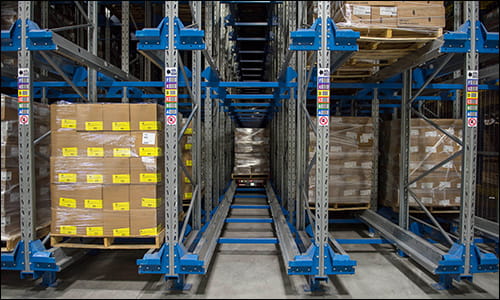The image depicts an interior scene of a warehouse, showcasing a detailed storage system made up of grey metal shelving units and rails. These metal structures are complemented by striking blue cross beams, with some components like the end caps also in blue, adorned with stickers that feature various colors including blue, purple, pink, yellow, orange, and green, along with arrows pointing to the left. The system consists of two rows and five columns of these shelves, prominently holding multiple parcels. The left side features two brown parcels, while the right side displays three more parcels, two at the bottom and one on top. A distant parcel is also visible in the center. These parcels are securely wrapped in a cling or cellophane-like wrap, hinting at a secure storage method. The grey-colored ground contrasts with the dark ceiling, completing the utilitarian architectural elements of this warehouse interior.